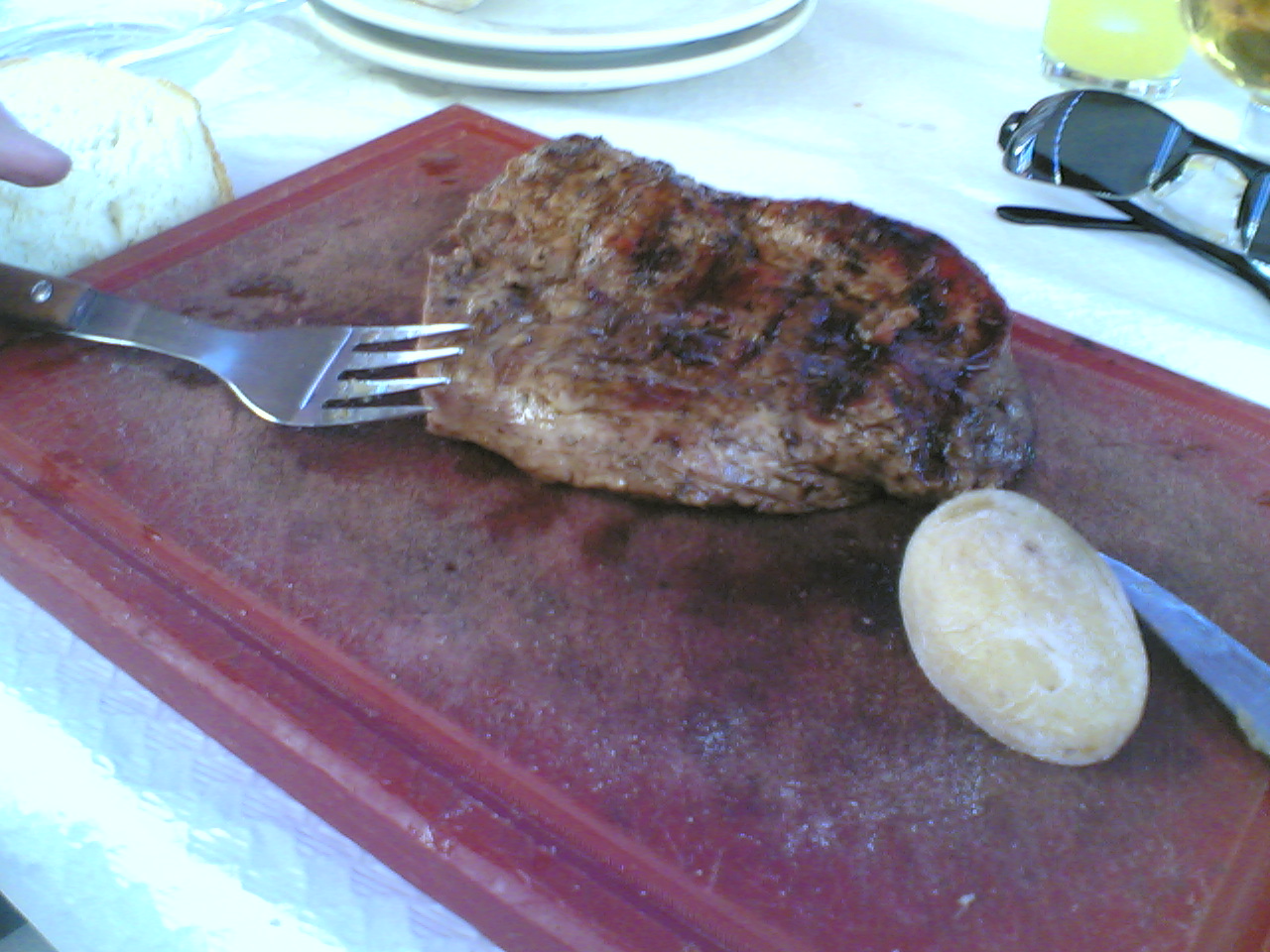The photograph captures a detailed moment at a carving station set on a table with a white tablecloth. Central to the image is a well-done, large steak with a seared top, resting on a worn red cutting board infused with numerous grooves. Beside the steak lies a round, powdered item which could either be a peeled potato or a small loaf of bread dusted with flour or sugar. In the top right corner of the cutting board, a large fork and steak knife await the next cut. Adjacent to these items, a pair of black sunglasses adds a casual touch to the scene. The table also features two stacked white plates and a glass of yellow liquid, enhancing the sense of an anticipated meal. Additionally, a finger is pointing into the picture from the top left corner, suggesting someone is mid-conversation or providing direction. This vibrant and bustling setup is accentuated by the hues of red, brown, black, gray, tan, yellow, and white.